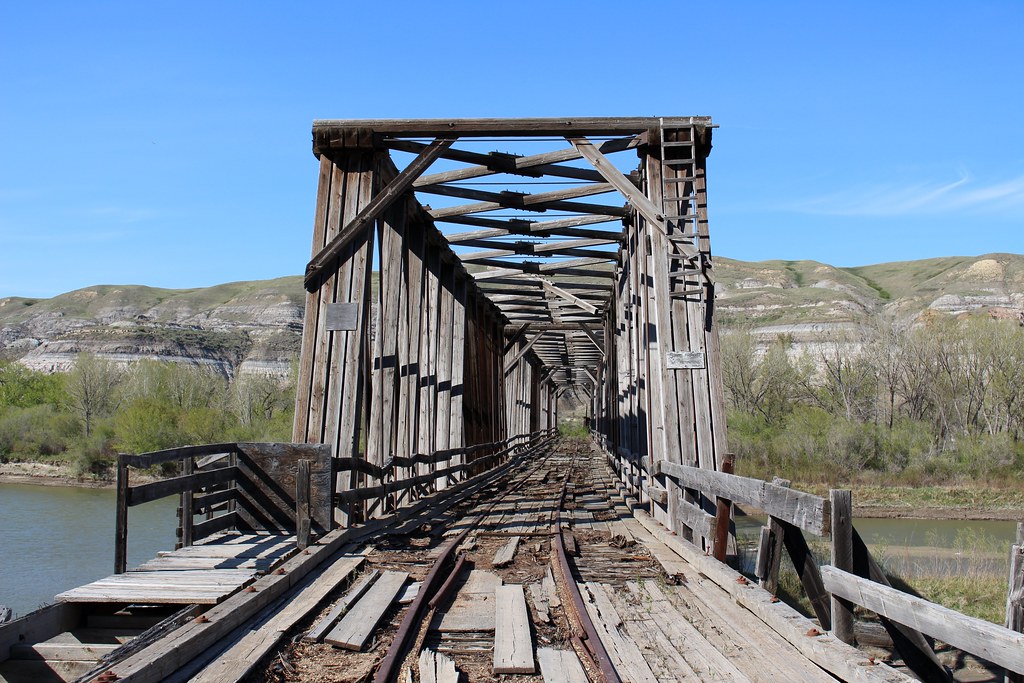This photograph captures an abandoned, decaying wooden railway bridge spanning a wide, flowing river with clear, bright blue skies above. The perspective of the image is down the length of the bridge, revealing rusted rails and rotting, scattered boards, suggesting that it hasn't seen a train in a long time. The bridge features a structure of support beams, partially open at the top, and a metal railing on the side. There are remnants of the service area or access points, including a ladder and stairs, though most of these are in disrepair. In the background, rolling hills and small mountains rise beneath the vast sky, and along the riverbank, lush green trees add to the serene yet neglected scene. The sunlight illuminates the weathered details of the bridge, casting shadows and highlighting the age and abandonment of this vintage railway trestle. The setting conveys a sense of history and quiet desolation.